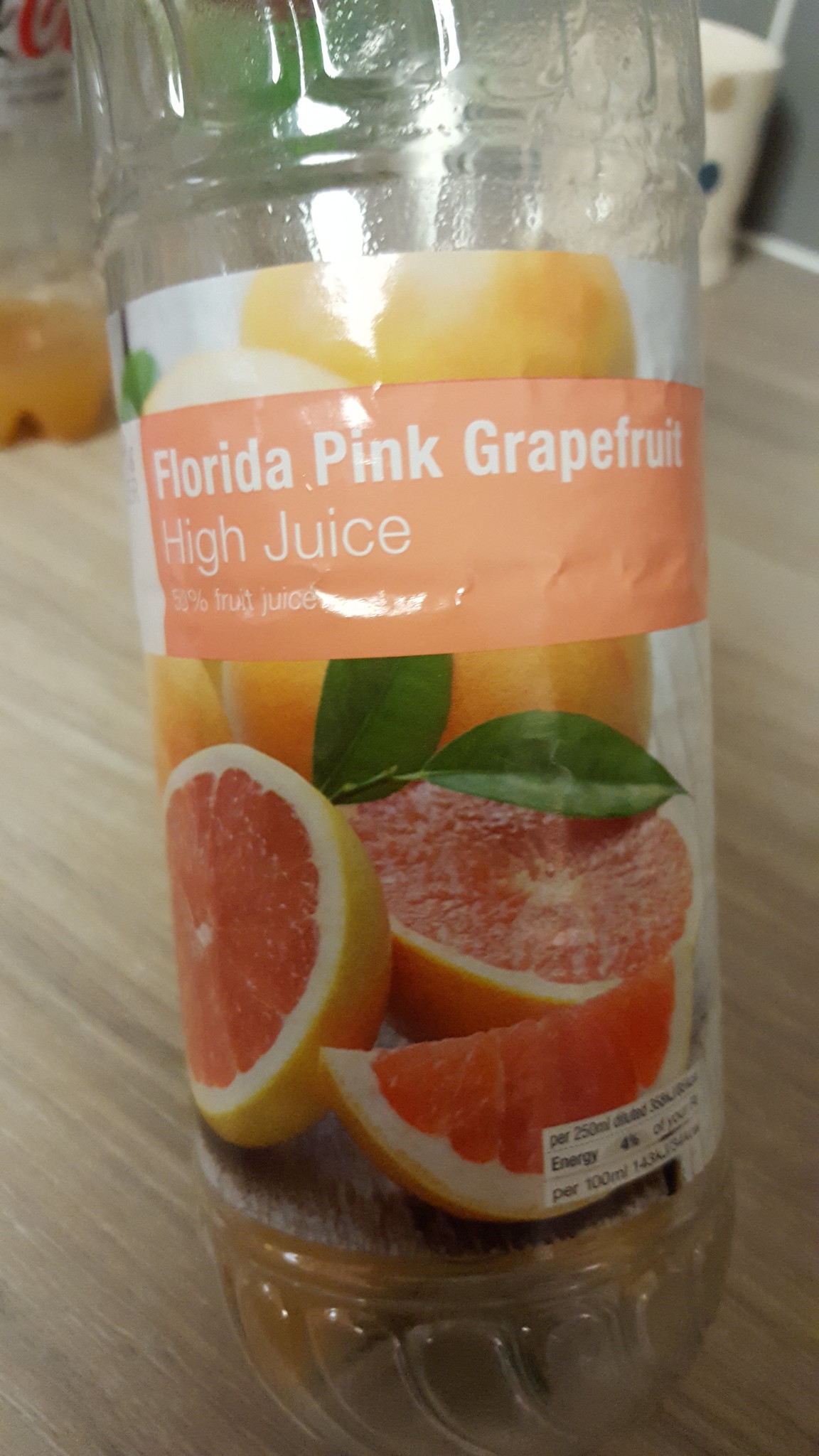In the image, prominently featured in the center, is a clear plastic bottle branded as "Florida Pink Grapefruit High Juice," indicating it contains 50% fruit juice. The bottle's label showcases vibrant images of citrus or orange slices adorned with two fresh green leaves. This bottle rests atop a rustic wooden table. 

To the top left of the image, there is a partially visible Coca-Cola bottle that has likely been reused; it contains a small amount of what appears to be orange juice, and the distinct shape and slight remnants of the label suggest it was originally a Diet Coca-Cola transparent bottle. 

On the top right, behind the grapefruit juice bottle and slightly obscured, is a white cup featuring a faint decorative pattern of gold and blue dots. The backdrop of the scene is composed of grayish tiles, serving as the wall, adding a subtle texture to the background.